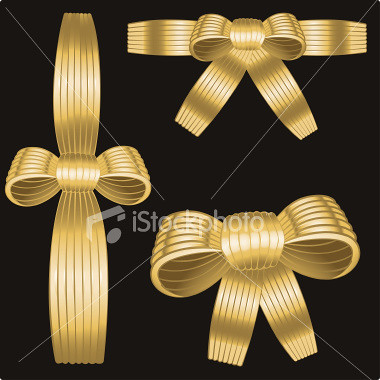This image features a black background adorned with three intricately designed gold bows, each crafted from ribbon with darker gold stripes. A crisscross watermark overlays the center, accompanied by the text "iStockPhoto" in white letters. 

In the upper right corner, the bow presents one loop pointing left and another right, anchored by a smooth center piece. From this, two tails extend outward to the sides, and two more tails cascade downward in a slightly more elaborate fashion.

The lower right corner displays a more traditional bow with a right and left loop and a smooth center, from which two ribbon tails extend downward at five and seven o'clock positions.

On the left side of the image, a vertically oriented bow features a simpler design, with a loop on either side of a smooth center, its tails extending vertically from top to bottom.

Overall, the image is a digitally crafted portrayal of gold ribbons on a strikingly dark canvas, marked by geometric watermarks and branding text.